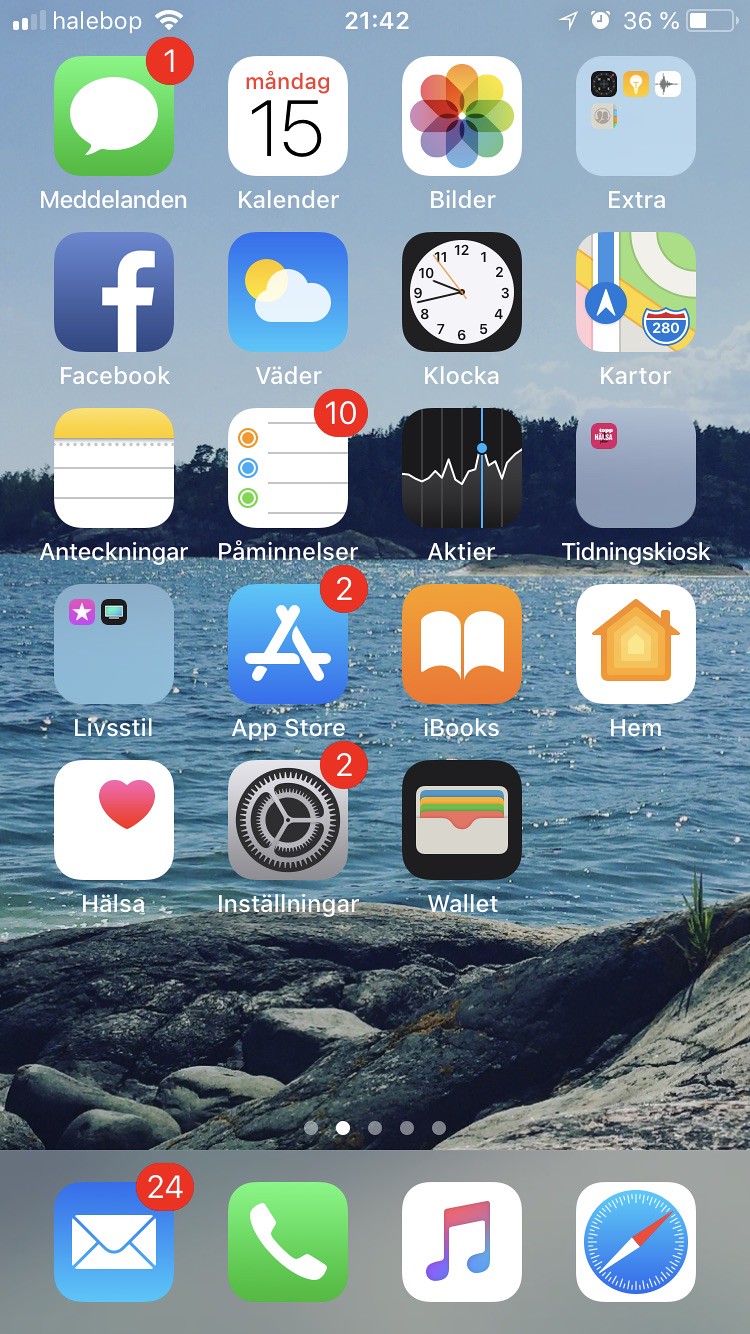This image appears to be a screenshot of an iPhone home screen. The device shows two bars of cellular service with "Hail Bop" written at the top, possibly indicating carrier information in another language. The phone has full Wi-Fi connectivity and displays the time in a 24-hour format, showing 2142 (9:42 PM). The battery level is at 36%, and an alarm has been set, with location services active.

On the home screen, the message app has one unread notification. Visible apps include Calendar, Photos, and a folder labeled "Extra." The user has several commonly used apps such as Facebook, Weather, Clock, Map, Notes, Reminders, and Stocks. Additionally, there are two folders with titles in different languages, indicating a multilingual interface. While some app names are in English, like Facebook, many are in another language. Other English-labeled apps include the App Store, iBooks, and Wallet. 

At the bottom dock, the prioritized apps are Mail, Phone, Music, and Safari. The background of the home screen is a serene image depicting a waterfront scene, adding a calming aesthetic to the display.